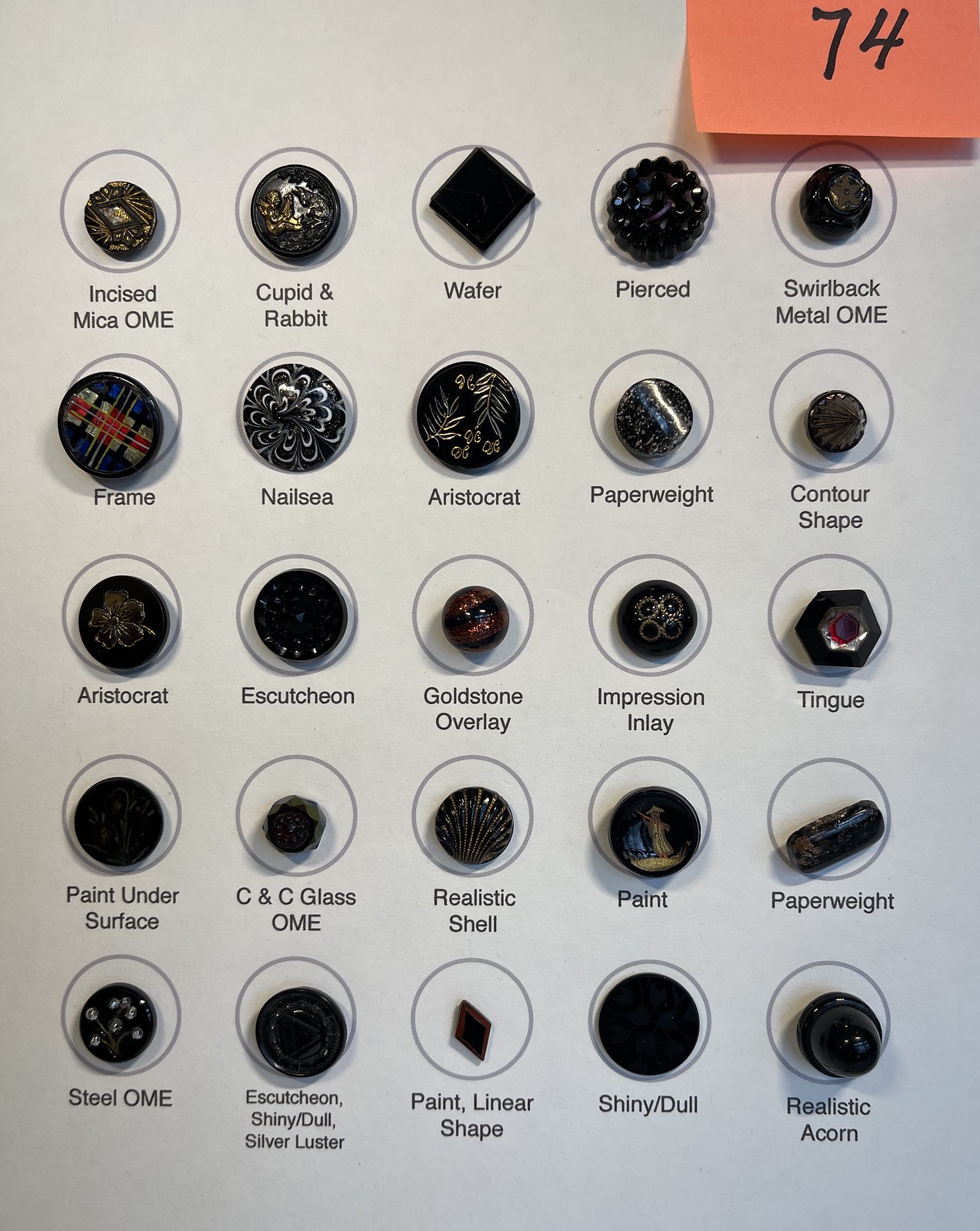The image depicts a white cardboard sampler card meticulously showcasing a collection of 25 elaborate buttons, arranged in a grid of five rows and five columns. Each button is housed within a circle and is intricately designed, featuring a range of materials and embellishments including jeweled, carved, translucent, and simple designs. Most buttons are predominantly black with ornate gold accents and various color embellishments. Each button has a corresponding label beneath it, providing a detailed description of its design. Notable buttons include "Insize Mica OME," which has a jewel embedded in it, and "Cupid and Rabbit," which features an engraving of a Cupid angel and a rabbit. Other labels include "Wafer," "Pierced Swirlback Metal OME," and "Frame," the latter being particularly colorful with shades of blue, white, red, and yellow. A yellow sticky note with the number "74" is affixed above the grid, adding an additional point of detail to this highly organized assemblage of decorative buttons.